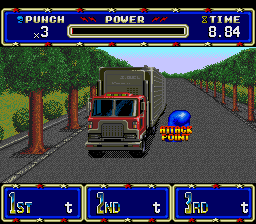The image is a computer-animated screenshot from a video game featuring a very large semi-truck, with a red cab and gray trailer, driving towards the viewer on a tree-lined road. The road is flanked by rows of green, rounded trees with brown trunks, reminiscent of an orchard. At the top, the interface displays key game information: "PUNCH x3" on the left, "POWER" in the center above a black rectangular object, and "TIME 8.84" on the right. In the center of the image, a blue object labeled "attack point" is positioned near the semi-truck. Along the bottom, three blue rectangular boxes labeled "first 1ST T", "second 2ND T", and "third 3RD T" span across the screen, indicating different game positions or options. Overall, the scene blends detailed visuals with crucial gameplay statistics for an immersive gaming experience.